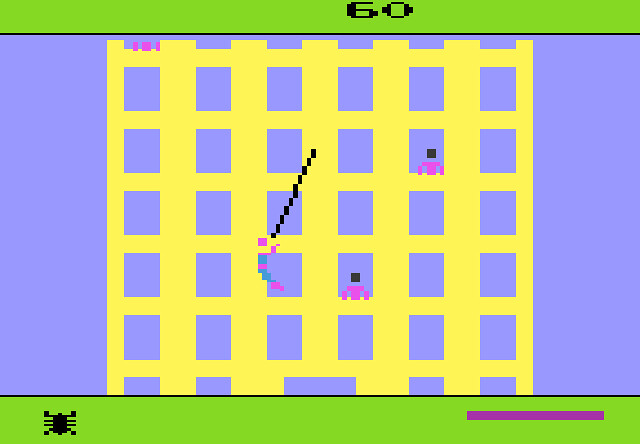A vibrant scene from a video game is depicted, showcasing a complex and colorful layout. At the top, there's a green rectangle displaying the number "60" in bold black text. On the bottom left of the image, a small bug is visible, contrasting against the overall design. The bottom right corner features a distinct purple bar. 

The main section of the image reveals an immersive video game environment set against a blue sky. Central to the layout is a yellow structure with multiple windows revealing the blue sky in the background. The structure is elaborately detailed with seven prominent yellow pillars, of which the central five are notably thicker. Purple squares are situated at the top level of the structure, possibly indicating figures peeking over the edge.

Horizontal bars run across the entire structure, adding to the intricate design. Within the windows, a purple figure is seen swinging on a black stick, while other windows display what appears to be characters with purple bodies and black heads. The entire scene is rendered in a pixelated style, creating a simple yet visually engaging lattice of colors and shapes.